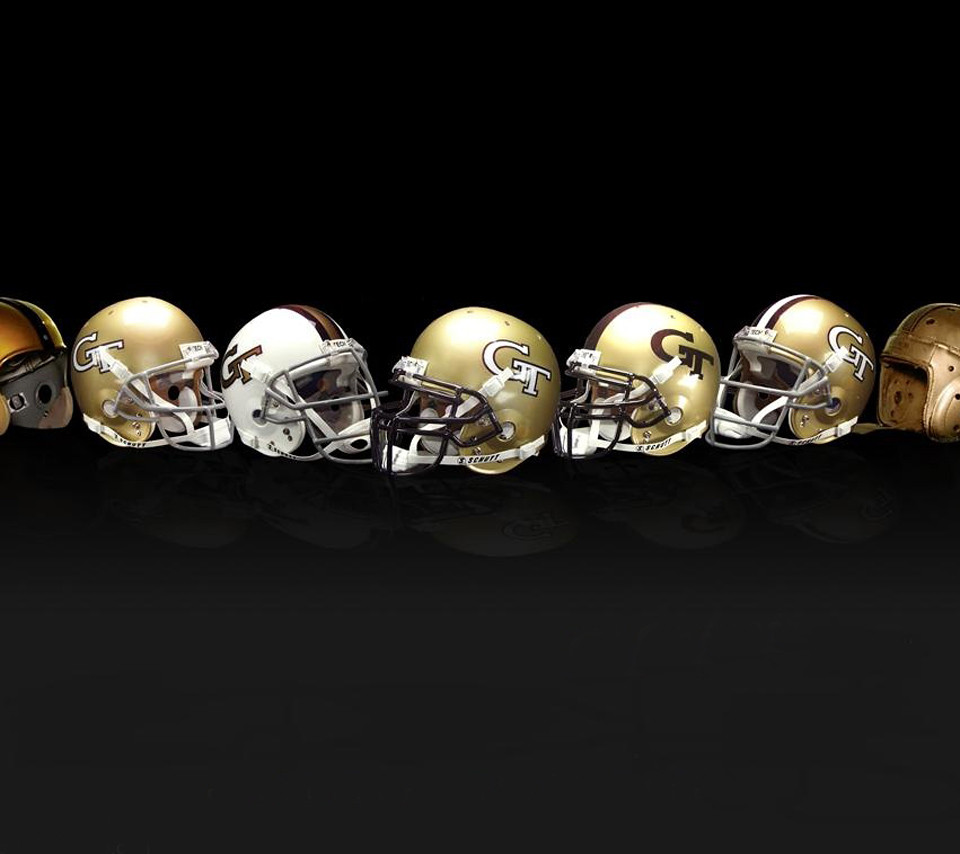The image showcases a row of seven football helmets arranged side by side against a black square background, approximately three-fifths of the way up the photograph. The central five helmets are modern with metallic face grills, while the ones on the far left and right are archaic leather helmets, lacking face protection. The helmets predominantly feature a gold, brown, and white color scheme and display a stylized "GT" logo on their sides. Notably, the first helmet on the far left has a vintage design with a brown top and black stripe, and the last one on the far right is another old design, appearing well-worn and entirely brown. In the faintly reflective surface beneath them, the helmets cast a subtle, transparent shadow.